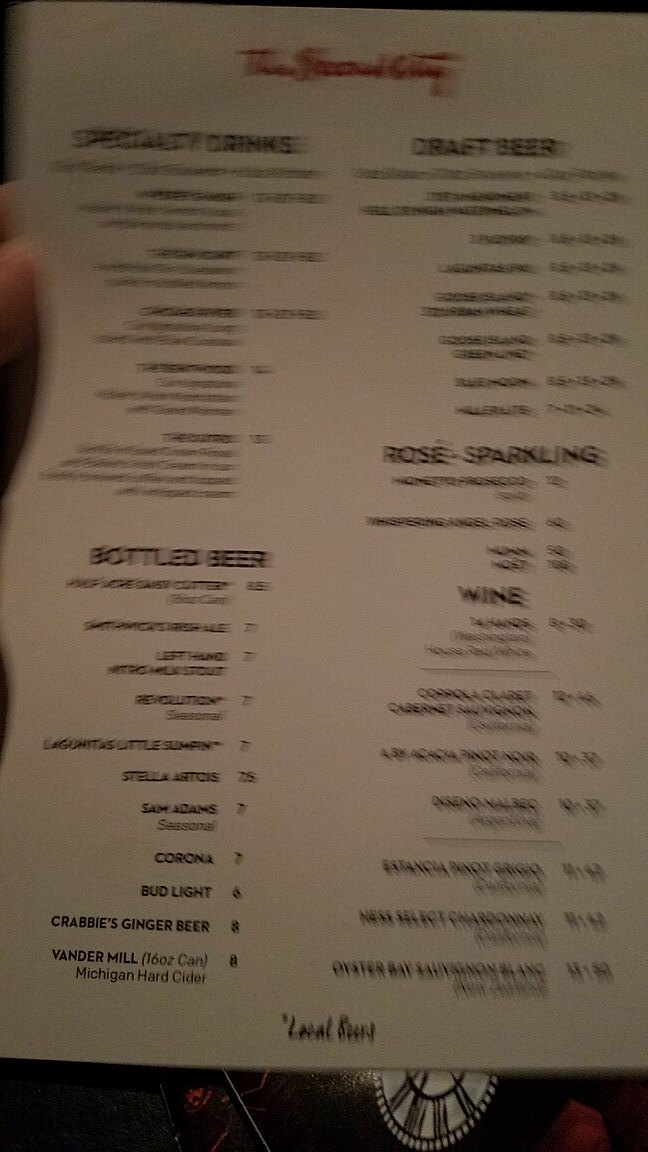**Image Description: A Fuzzy Snapshot of a Drink Menu**

In this blurry photo, a hand is partially visible in the top left corner, suggesting someone might be holding the menu. The menu itself is printed on white paper with bold red writing at the top, which is difficult to decipher but might indicate the name of the restaurant or the city it is located in. The primary focus is on the various categories of drinks offered, with large, bold headings such as "Specialty Drinks," "Draft Beer," "Bottled Beer," and "Rosé-Sparkling" clearly visible despite the overall haziness.

Beneath the heading "Bottled Beer," some details are legible. Listed are:

- **Corona** priced at **$7**
- **Bud Light** at **$4**
- **Sam Adams**
- **Stella Artois**

Due to the poor image quality, prices for Sam Adams and Stella Artois cannot be determined, and several other entries under this category are unreadable.

The bottom of the menu is adorned with a line of text in a different font, stating "Local something," but the exact wording remains unclear. Interestingly, an object resembling a clock face with black Roman numerals on a white background spans the width of the image at the bottom, though its purpose or connection to the menu is ambiguous.

Overall, the image captures a lengthy drink menu that is mostly illegible, save for a few key headings and drink names.